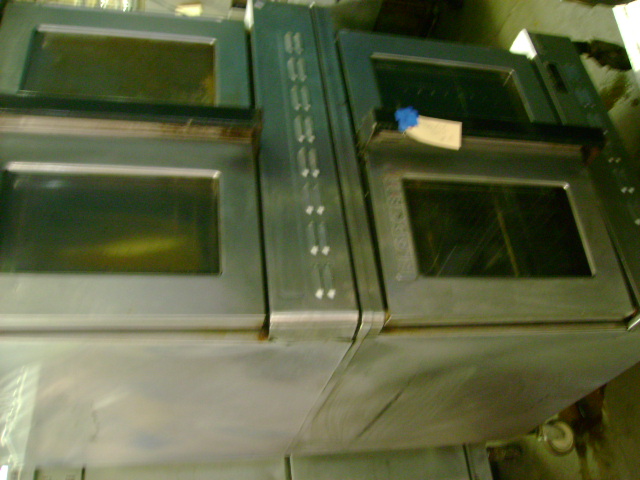This photograph, although out of focus and oriented sideways, showcases an old piece of industrial equipment, likely an oven or perhaps a refrigerator, characterized by its robust metal construction. The equipment rests on a metal cart with castered wheels, adding to its mobility. It features four glass-paned doors, arranged in upper and lower sections, allowing visibility into its interior. The doors have vertical handles that extend along their length. The metal surface shows signs of age, with noticeable rust. A white tag with blue details is affixed to the handle of the bottom door. The background reveals a concrete floor and a suggestive silver wall, adding to the industrial ambiance. Overall, the image’s color palette leans towards OD green and grayish hues, contributing to a dull, worn-out aesthetic. Although blurry, the photograph hints at a functional yet antiquated and weathered piece of equipment, standing ready for inspection.